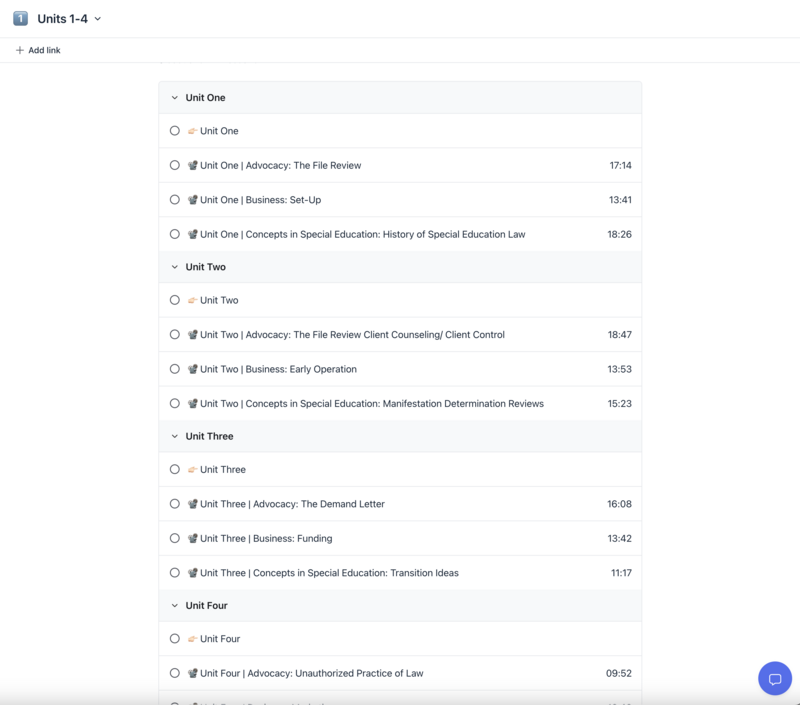This is a screenshot from an unidentified source displaying a list of units and their corresponding topics, organized into four main categories. At the top, there is an option labeled "Add Link." The units are as follows:

- **Unit 1:**
  - **Advocacy:** "The File Review" (1714)
  - **Business:** "Setup" (1341)
  - **Concepts in Special Education:** "History of Special Education Law" (1826)

- **Unit 2:**
  - **Advocacy:** "The File Review: Client Counseling/Client Control" (1847)
  - **Business:** "Early Operation" (1353)
  - **Concepts in Special Education:** "Manifestation Determination Reviews" (1523)

- **Unit 3:**
  - **Advocacy:** "The Demand Letter" (1608)
  - **Business:** "Funding" (1342)
  - **Concepts in Special Education:** "Transition Ideas" (1117)

- **Unit 4:**
  - **Advocacy:** "Unauthorized Practice of Law" (952)

The image contains no photographic elements or visual depiction of people, animals, birds, plants, flowers, trees, buildings, or automobiles.